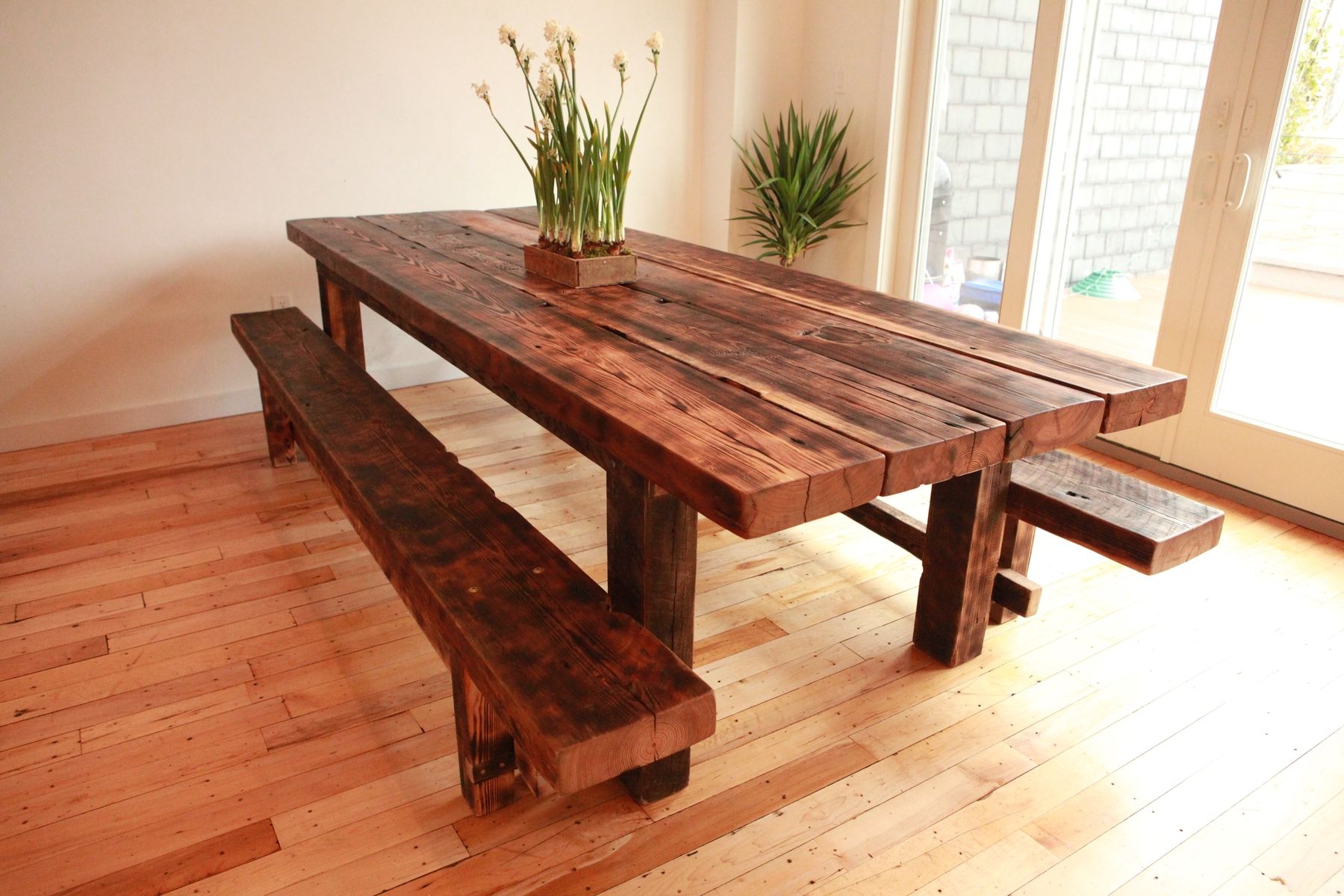The image is a horizontal rectangular photograph taken inside a house, showcasing a prominent handmade picnic table crafted from dark wooden planks. This sturdy, long picnic table features attached benches on either side, mimicking the style of tables typically found in parks. The table is positioned on a wooden floor, and the only item adorning its surface is a round vase containing a plant with what appear to be white flowers. The room is bathed in abundant natural light streaming through large French doors, which are cream-colored and open outward to a patio. These doors have visible door handles. In the corner of the room, another plant adds a touch of greenery. The walls of the room are also painted in a matching cream color, complementing the overall light and airy feel of the space.